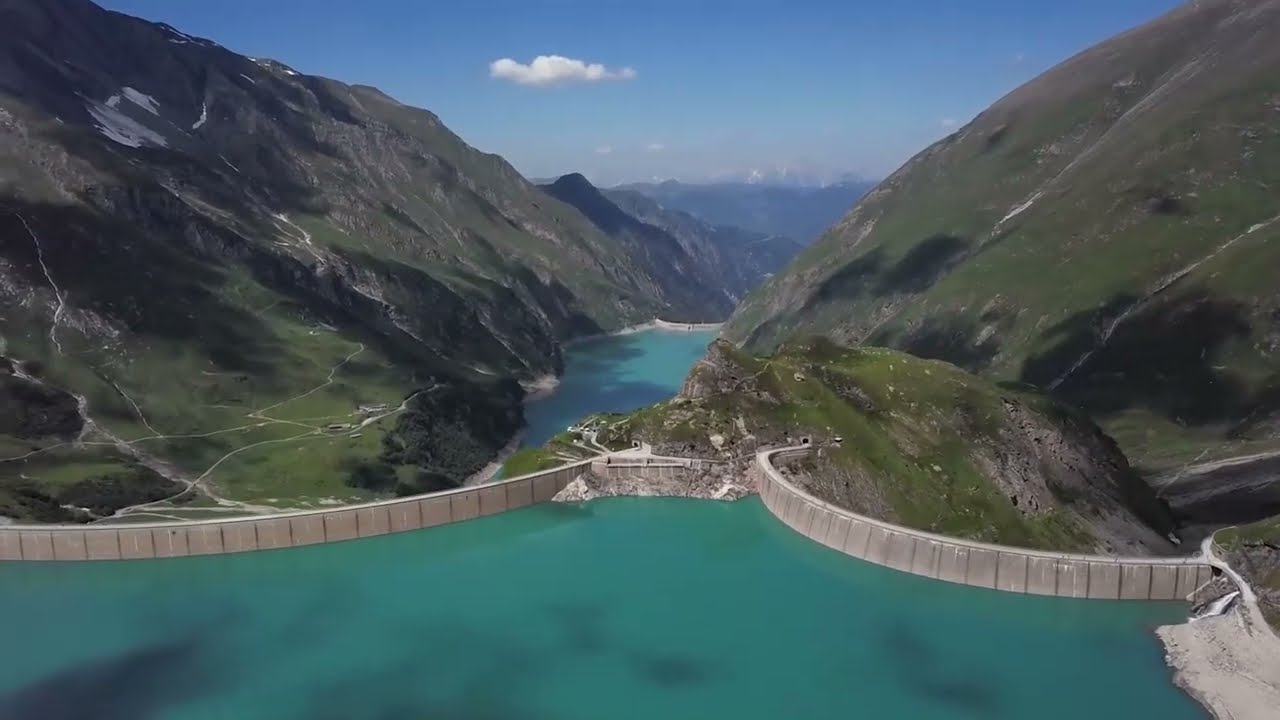The image is an impressive aerial photograph capturing a dam situated in a picturesque, mountainous region. From an elevated perspective, likely from a helicopter or a plane, we see this curved, green-colored dam positioned prominently in the center. On the lower half of the photo, a vast reservoir stretches out, filled with stunning turquoise blue water. Above the dam, the river continues to flow, its blue waters contrasting with the contained reservoir below. Flanking both sides of the river are grand mountains, their surfaces lush with green grass and dotted with rocks. The clear blue sky overhead is punctuated by scattered clouds, which cast soft shadows over the mountains, adding depth and dimension to the scene. The dam itself features a substantial barrier that appears robust enough to permit walking or driving, possibly extending into tunnels within the mountains. Overall, the image beautifully captures the harmonious blend of natural and engineered landscapes.